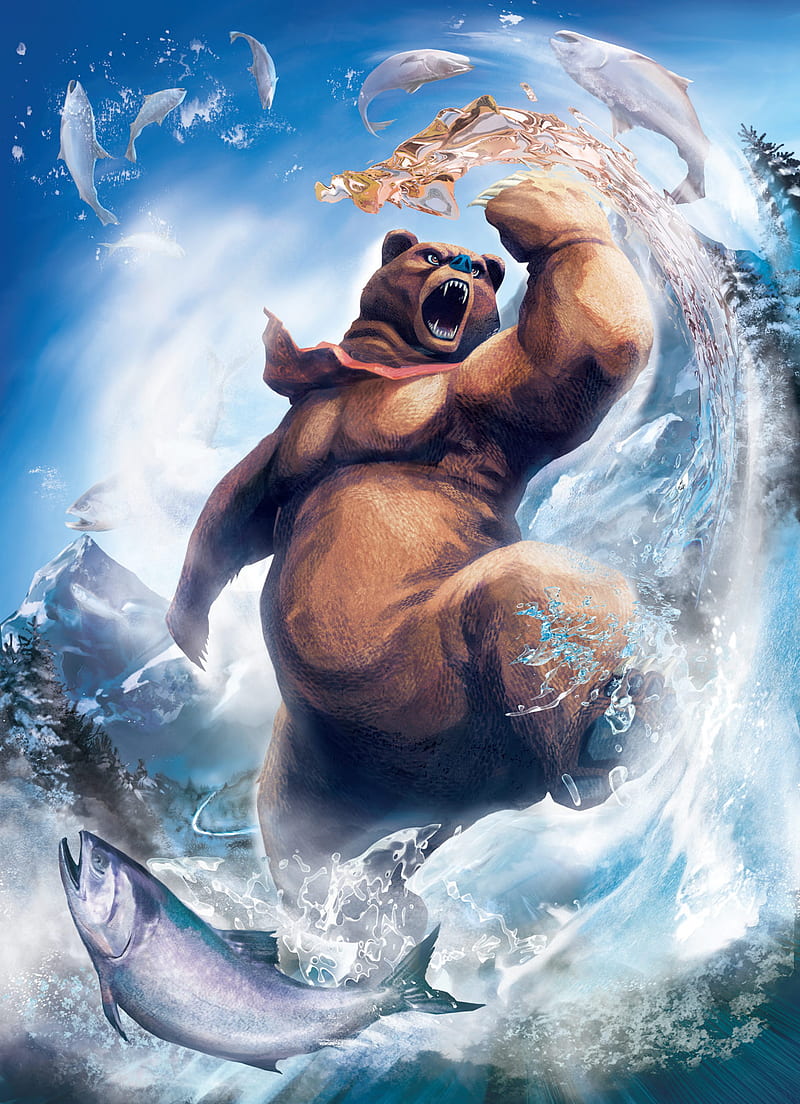In this computer-generated art poster, a ferocious brown bear is depicted in a dynamic scene set against a multi-shaded blue background. The bear, standing partially submerged in water, expresses sheer rage with its mouth wide open, baring sharp teeth, and eyes furrowed in anger. It's swiping its massive claw through the water, creating a dramatic splash that sends droplets flying into the air, while its other leg stomps into the river, emphasizing the motion. The water around the bear churns violently, forming waves and shooting golden droplets above its head.

Several silvery fish, caught in the bear’s chaotic assault, whirl above and around him, with one notable fish swimming away in the bottom right corner as if it has narrowly escaped the bear’s grasp. Another fish is seen leaping out of the water towards the viewer. The fish appear almost spiraled in the air, accentuating the bear's vigorous movement.

Around the bear’s neck is an enigmatic, tube-like object, possibly an AI-generated error, adding a strange twist to the artwork. The background features a picturesque landscape with a blue sky, scattered clouds, towering mountains to the left of the bear, and snow-covered trees to the right. A particular tree near the bottom left blends with the water splashes, adding depth to the scene. Overall, this detailed and action-packed portrayal captures the raw power and frustration of the bear in its natural habitat.